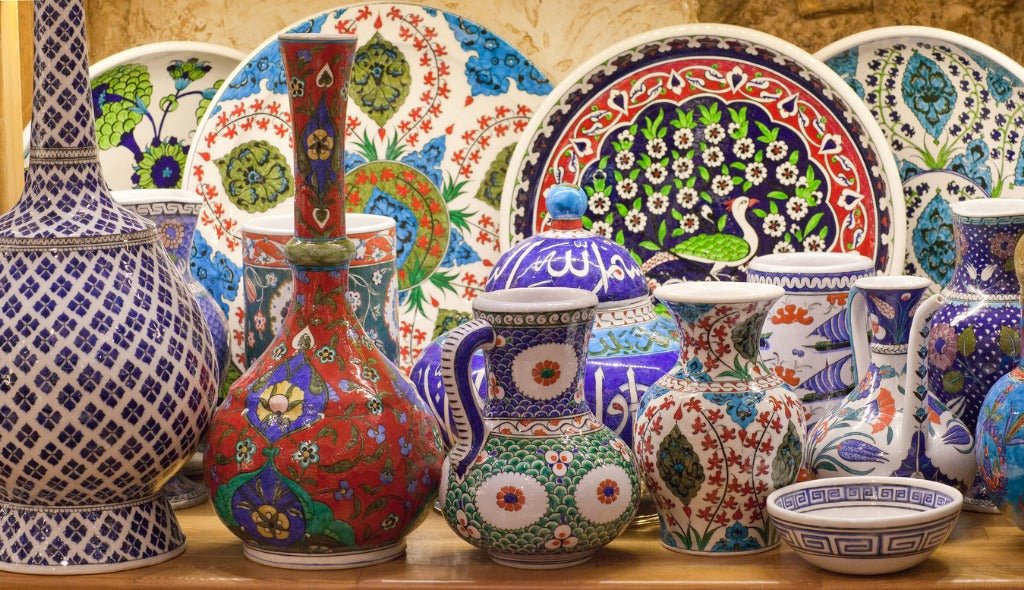The photograph showcases an elaborate display of various ceramic pieces, all meticulously arranged side by side on a table. The collection includes vases, pitchers, goblets, and small bowls, each decorated with intricate and colorful patterns. At the forefront, there’s a pitcher adorned with white circles, while to its left stands a taller, red pitcher with a slender neck. Further left, an even larger red pitcher features striking blue diamond patterns. A prominent vase on the far left exhibits a repeating grid of cross shapes or squares, with intricate floral motifs and a bird amidst green leaves at its center.

In the background, several large, round plates and serving platters are leaning against a brown wall, creating a layered effect. One notable plate features a green feathered bird surrounded by delicate white flowers. The overall design of the ceramics appears to draw inspiration from tribal and Aztec styles, with an array of blue squares, red, yellow, and green floral patterns, and other colorful geometric designs. The lighting in the photo casts shadows to the left, suggesting the light source originates from the right side. This detailed and vivid arrangement reflects a rich cultural artistry, reminiscent of Russian, Polish, and Aztec influences.